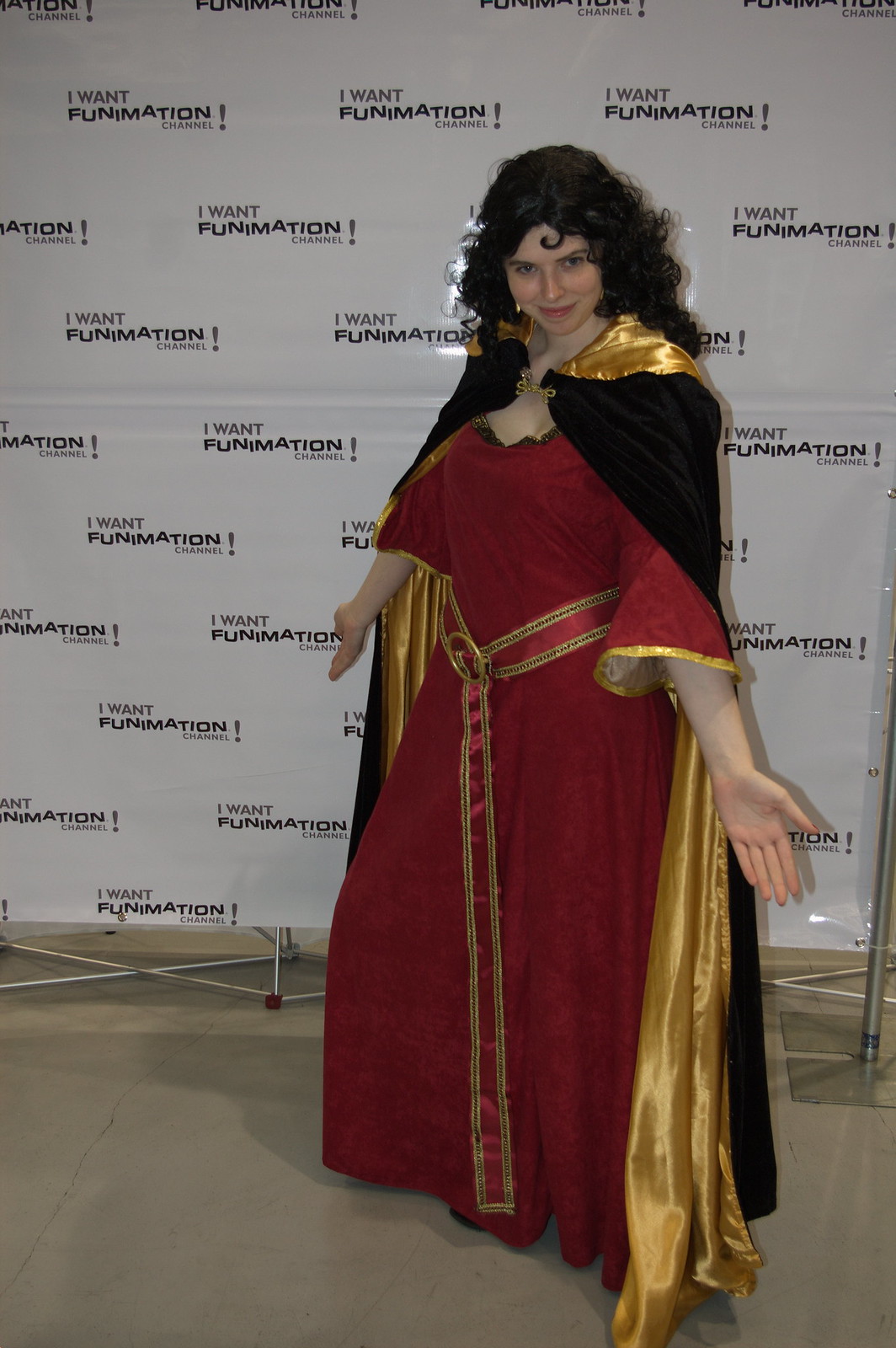The photograph captures a woman dressed in an elaborate royal-like outfit, posing with both hands extended to her sides. She wears a long, flowing red silk dress adorned with a gold and red belt that drapes nearly to the floor, complemented by a black cape with a gold interior clasped around her neck. Her dark, curly hair cascades gracefully on either side of her face, framing her expressive smile accentuated by lipstick. Behind her, a white banner repetitively displays the phrase, "I want Funimation Channel." The scene appears to be set on a concrete floor, suggesting it was taken indoors, likely at a convention such as an anime event. Her arms are held out, with palms facing outward, adding a dramatic flair to her regal pose.